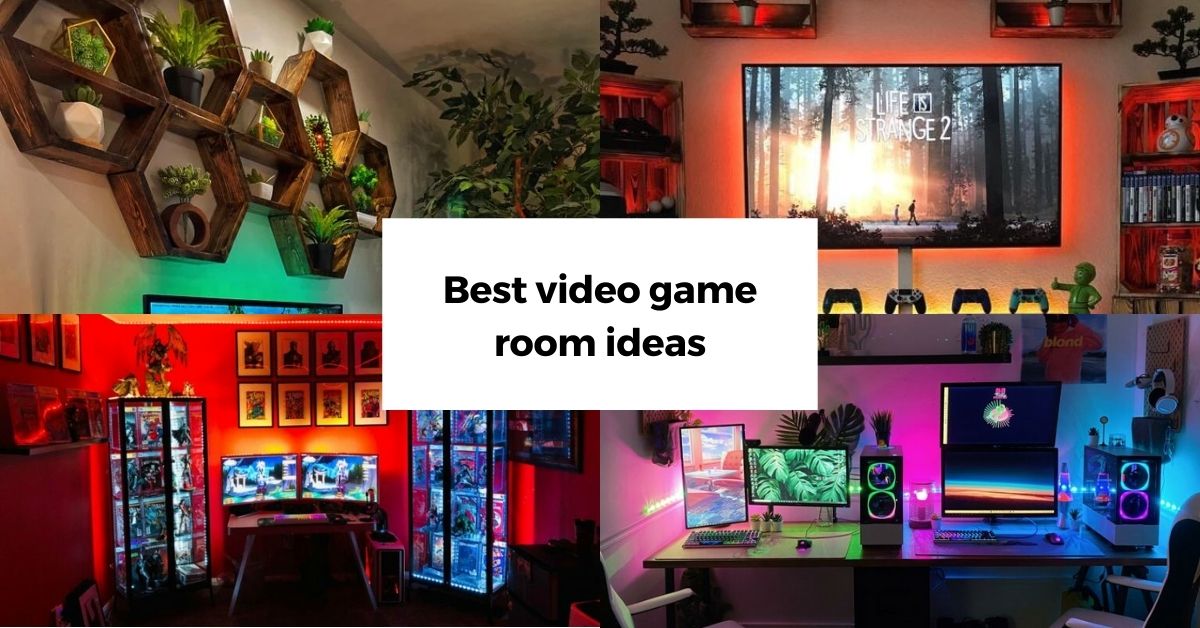This image is a collage of four distinct video game room setups, presented in a widescreen layout with the overall image divided equally into four quadrants. Each quadrant showcases a uniquely themed room design. At the center of the collage is a prominent white box that partially obscures each quadrant and features the text "Best Video Game Room Ideas" in bold black ink.

- **Top Left Quadrant:** This room has a lush jungle theme, characterized by green lighting emanating from the top of a partially visible TV screen. The wall features wooden hexagonal paneling adorned with various plants and includes a substantial, tree-like plant extending towards the ceiling, enhancing the natural aesthetic.
  
- **Top Right Quadrant:** This section presents a sleek and modern setup centered around a wall-mounted TV, with red ambient lighting creating a striking backdrop. Below the TV, a row of game controllers is neatly lined up, and bookcases flanking either side are filled with games or DVDs. Additionally, a Pip-Boy statue from Fallout adds a touch of gaming culture.

- **Bottom Left Quadrant:** This room is bathed in intense red lighting and features a double screen setup on a desk. The walls are decorated with an array of photos arranged in a precise grid pattern. Glass cabinets illuminated by LED strips flanking the desk add a modern touch and display various items or collectibles.

- **Bottom Right Quadrant:** This setup boasts a wide desk equipped with two computers side by side, each with multiple screens in both vertical and horizontal orientations. The room is illuminated by multi-colored lighting from the tower computers and the backs of the monitors. Two chairs are positioned side by side, indicating a cooperative gaming environment. 

Each quadrant in this collage provides unique inspiration for video game room designs, ranging from natural themes to intensely lit modern setups, catering to a variety of aesthetic preferences.